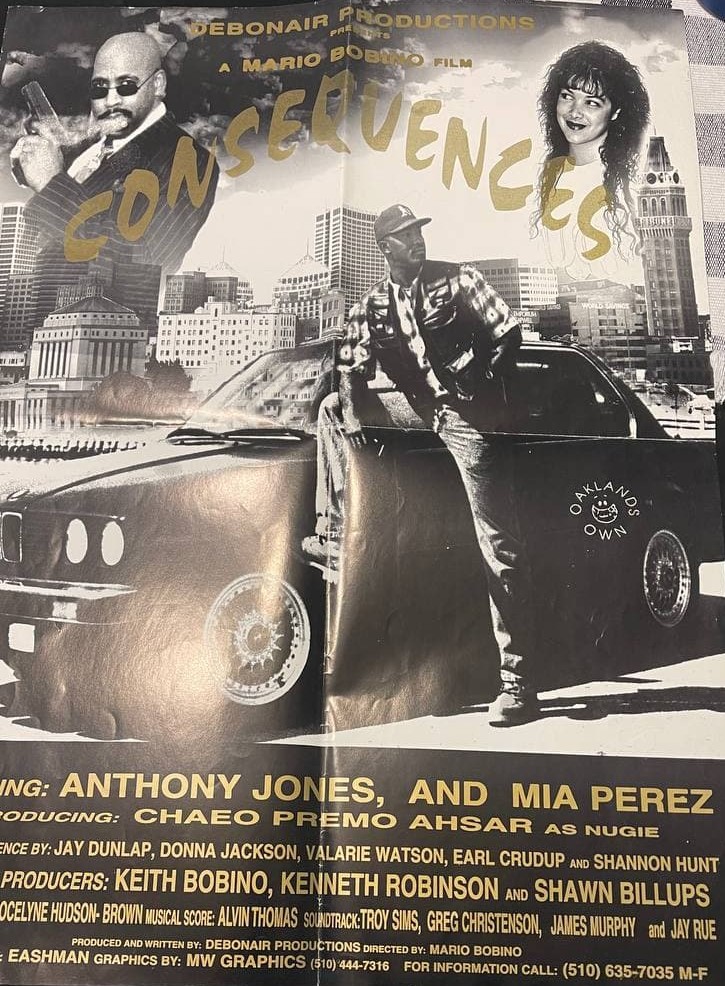The movie poster for "Consequences," a film by Mario Bobbino presented by Debonair Productions, features striking gold text at the top that reads, "Debonair Productions presents a Mario Bobbino film." Dominating the central graphic is an African-American male leaning against a vintage BMW, with the car’s passenger side displaying the logo "Oakland's Own," suggesting a California setting. This visually arresting, black-and-white poster has a creased look, as if folded into quarters. 

On the left side of the poster, a bald African-American man with a mustache and sunglasses, clad in a pinstripe suit, holds a gun up in the air. The right side features a young Latina woman with long, curly hair, casting a flirty glance and a half-smile at the armed gentleman. Behind her, there is a backdrop of a cityscape that heightens the urban atmosphere of the poster.

At the bottom of the poster, the names of the film's stars—Anthony Jones, Mia Perez, Cheo Primo, and Asar (as Nugi)—are prominently displayed, along with a list of other contributing artists, though some of these names are partially cut off due to the poster's folding.